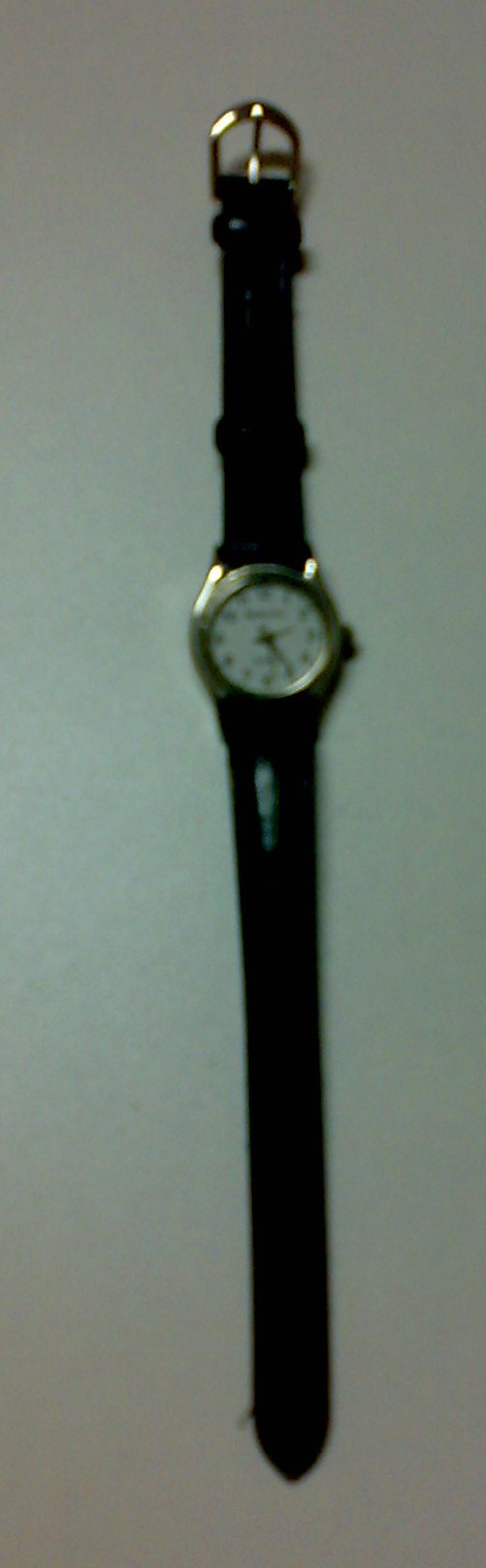This vertical, narrow, and slightly blurry image showcases a woman's analog wristwatch, photographed with the strap extending from the top to the bottom of the image. The watch, a potential Timex with a classic design, features a small white face encircled by a gold-tone bezel. The current time displayed is approximately 2.24. The wristwatch, equipped with a black or dark brown leather strap, also includes a gold-tone buckle. The watch face is adorned with Arabic numerals and black minute and second hands. The entire setup is laid out on an unclear white surface. The image’s low resolution focuses primarily on the center of the watch, contributing to slight blurriness in finer details.